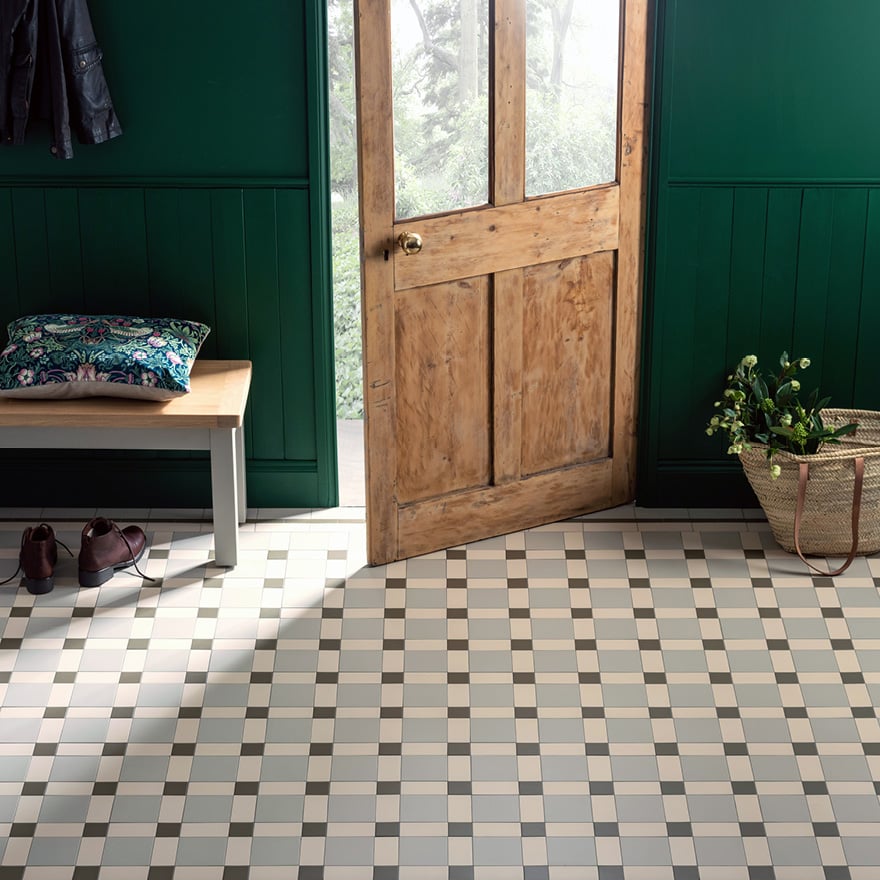Captured from a slightly elevated perspective, presumably from a staircase, the photograph showcases the interior entryway of a cozy, country-style home. The centerpiece is the partially open wooden door, adorned with two rectangular glass panes near its top, allowing slivers of light to filter through. The door reveals glimpses of an inviting outdoor scene with trees. Flanking the door is a small bench-like table to the left, upon which rests a green floral-print throw pillow. Beneath the bench lie a pair of brown leather Oxford-style shoes. Adjacent to the door on the right is a woven basket containing vibrant green plants. The walls are painted in a rich hunter green hue, adding warmth to the space, while the floor features a striking pattern of gray, dark gray, and white tiles arranged in a checkered design. Additionally, the room features wooden wainscoting harmonizing with the door's aesthetics, and a leather jacket hangs on the wall to the left, completing the picturesque, homely vignette.